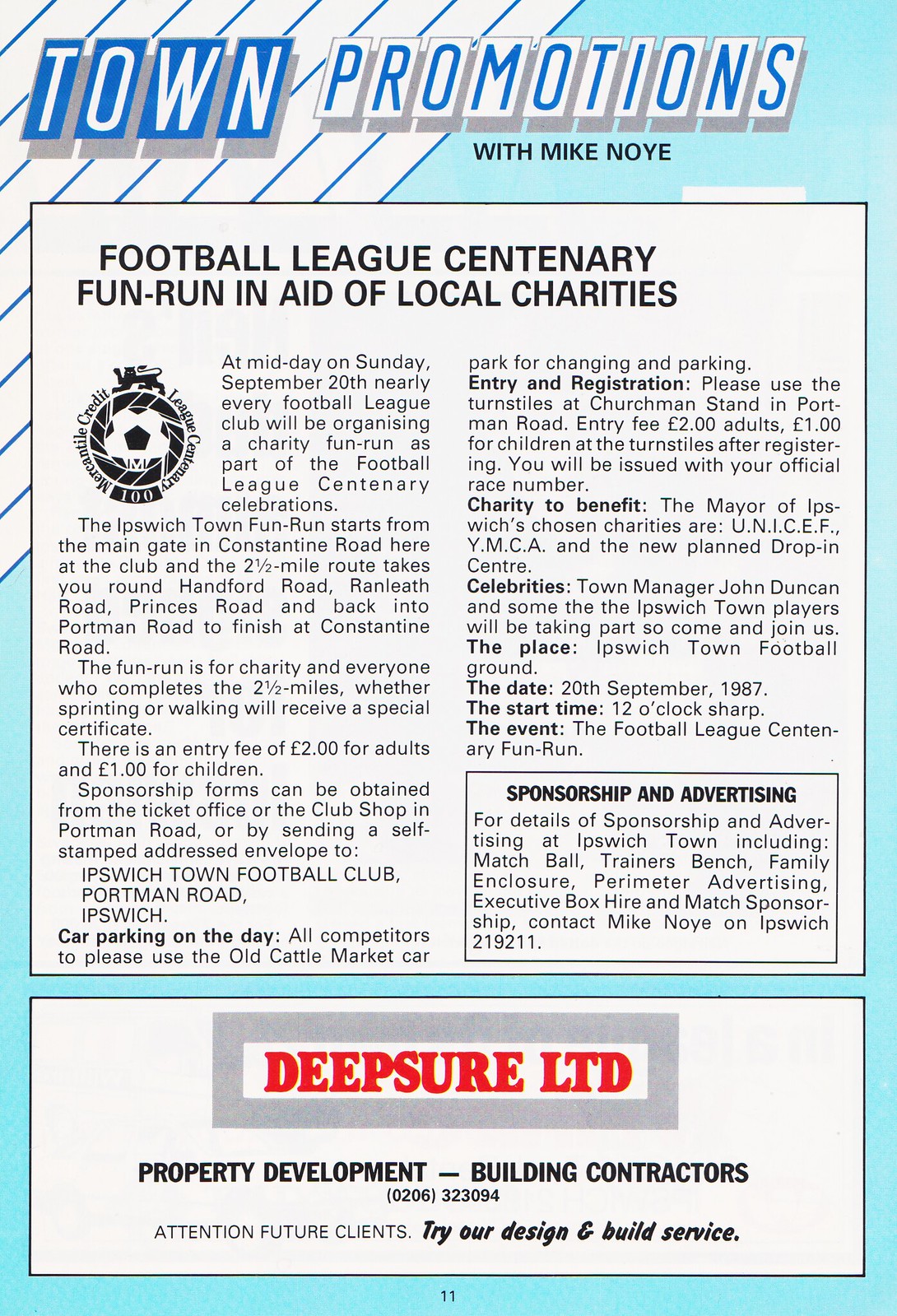The image is an advertisement titled "Town Promotions." At the top, "Town Promotions" is displayed in white text over blue, right-tilted background squares. The subtitle "Promotions" appears in blue text over white squares, set against a predominantly light teal background, with the upper left corner featuring a white section with diagonal blue lines.

Central to the ad is a large yellow-white box with multiple paragraphs detailing an event titled "Football League Centenary Fun Run in Aid of Local Charities." The event takes place at midday on Sunday, April 20, involving nearly every Football League club. Specifically, the Ipswich Town Run starts from Constantine Road, covering a 2.5-mile route via Hartford Road, Leith Road, Princess Road, and Portman Road, finishing back at Constantine Road.

The text in this section includes bolded headers like "Car Parking on the Day," "Entry and Registration," "Charity to Benefit," "Celebrities," "The Place," "Date, Start Time, and Event," and "Sponsorship and Advertising," which provides sponsorship details and event logistics.

At the bottom of the image is another box with a white background and a gray rectangle behind it. "Deep Shore LTD" is prominently displayed in red text, followed by "Property Development - Building Contractors" in black text. Further details include a contact number, 0206-323-094, and a promotion for their design and build service, highlighting "Attention Future Employees." The number 11 is marked at the very bottom of the ad.